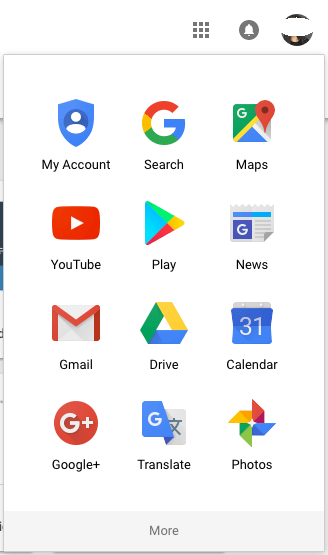A screenshot from a mobile device displaying a grid of application icons, each with their respective labels below. The icons are organized in four rows of three.

**Top Row:**
1. **My Account** - An icon featuring a shield with a basic person figure.
2. **Google Search** - A "G" in rainbow colors, identified as the Google Search app.
3. **Google Maps** - An icon of a map with a location marker (pin).

**Second Row:**
1. **YouTube** - A red square with a white play button centered.
2. **Google Play** - A rainbow-colored triangle, labeled as "Play."
3. **Google News** - An icon resembling a newspaper with a "G" on it.

**Third Row:**
1. **Gmail** - An envelope icon indicating the Gmail app.
2. **Google Drive** - A triangle composed of yellow, blue, and green segments.
3. **Google Calendar** - An icon representing a tear-off calendar page with the number "31."

**Bottom Row:**
1. **Google+** - A "G+" symbol, corresponding to Google Plus.
2. **Google Translate** - A "G" followed by a character in another language.
3. **Google Photos** - A multi-colored pinwheel icon.